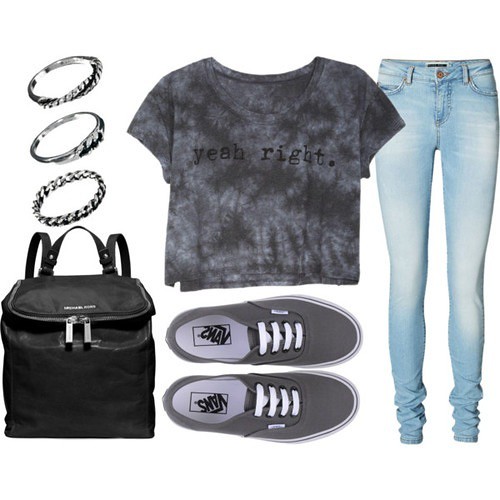The image showcases a stylish casual outfit laid out neatly, likely aimed at young women. At the center, there is a light gray and black tie-dyed T-shirt with black lettering that reads "yeah, right." Below the T-shirt, there is a pair of gray Vans sneakers with white soles and shoelaces; the left shoe has "Vans" printed backwards inside, while the right shoe has it upside down. On the right, a pair of light-colored blue skinny jeans are placed, slightly wrinkled at the bottom. To the left of the shirt, there are three silver, braided bracelets. Below the bracelets, a black backpack with silver zippers and white lettering across the top completes the ensemble. The items appear to be arranged either for an advertisement or to showcase a carefully curated collection.